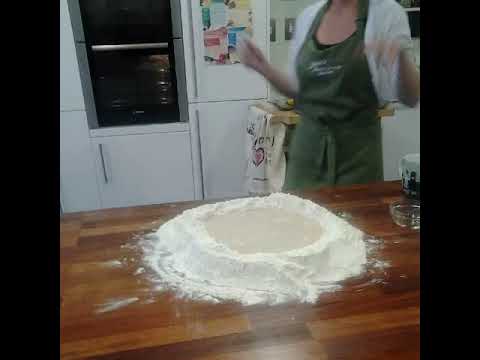In the image, a white woman, mostly seen from the shoulders down, stands in her white-appliance kitchen with a green apron over a light blue shirt. She is positioned slightly to the right of the center. Her arms are raised slightly, suggesting she is busy in the culinary process. In front of her is a large, smooth, wooden table composed of narrow, multicolored brown wooden slabs. The table hosts a giant, cylindrical mound of flour with additional flour scattered around it. Behind her, the kitchen features off-white cabinets with long metal handles, a black stove with metal trim, and a refrigerator covered with multicolored flyers and pictures. The image is cropped into a square with black bars on the left and right sides, emphasizing the central focal points of the woman, the flour, and the kitchen elements.